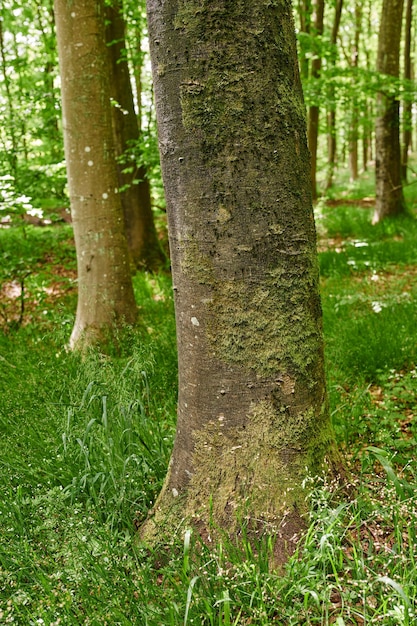This color photograph, in portrait orientation, features a large, majestic tree in a forest setting. The tree trunk, light brown and wide, extends from the ground to roughly a third of the way up, showcasing patches of light and dark green moss. Surrounding the tree are several additional large trees to the left, a few smaller ones to the right, and a stand of tall, slender trees in the background. The base of the tree, positioned near the bottom of the image, is encircled by lush green grass dotted with tiny flowers at the tips of the blades. Light filters through the canopy, casting a gentle, dappled sunlight across the scene, highlighting the verdant undergrowth and creating a tranquil, natural atmosphere indicative of a serene forest landscape.